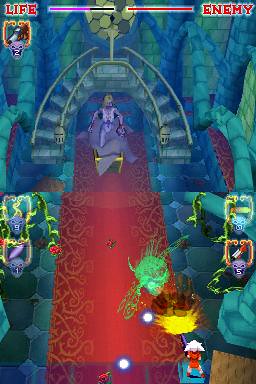In this image of a computer game screen displayed in portrait orientation, vibrant and colorful visuals dominate the scene. At the top of the screen, a red bar labeled "Life" is visible, while a label reading "Enemy" is positioned to the right. A small globe-like icon in green and gray leads downward, transitioning into a series of staircases. Descending the staircases is a man running on a red carpet. Scattered throughout the scene are various peculiar and indistinct creatures, suggesting a possible medieval battle setting. One prominent figure stands on a blue rug; this character has blonde hair, wears a red shirt, and a skirt-like garment that ends above his knees. In front of him, a blaze of gold adds to the intricate and detailed environment of the game, contributing to the overall complexity and visual appeal of the scene.